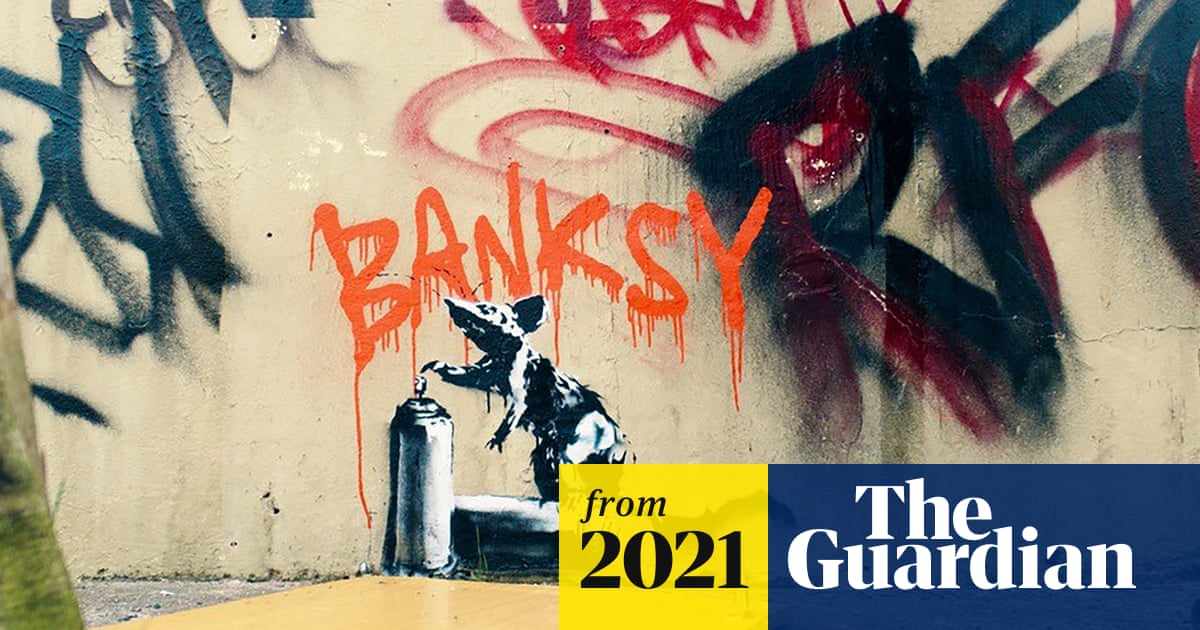The photograph showcases a piece of graffiti art on a beige, possibly light tan, exterior wall, attributed to Banksy. The artwork features prominently near the bottom of the wall, where the word "Banksy" is inscribed in orange, with paint dripping from each letter. Below this, a gray rat is depicted next to a cylindrical flask, appearing as if it's attempting to drink from it, styled in Banksy's signature black and white. 

The wall itself is older and cracked, adorned with additional graffiti. On the upper left corner, some large navy blue letters are partly visible but run off the edge of the picture. On the right side, the letters "RFO" are written in reddish black, accented by red smears. The left side features blue scratches or brushstrokes, adding to the chaotic aesthetic. Above these, there is another red-colored text.

In the lower left corner of the photograph, there is an inset with two distinct sections: a yellow background with black text reading "From 2021" and a blue segment with white text that says "The Guardian." This inset provides context to the graffiti’s origin and its subsequent feature in The Guardian newspaper. The setting of this piece is unmistakably street art, reflecting both the art form's transient nature and its impactful presence on urban landscapes.